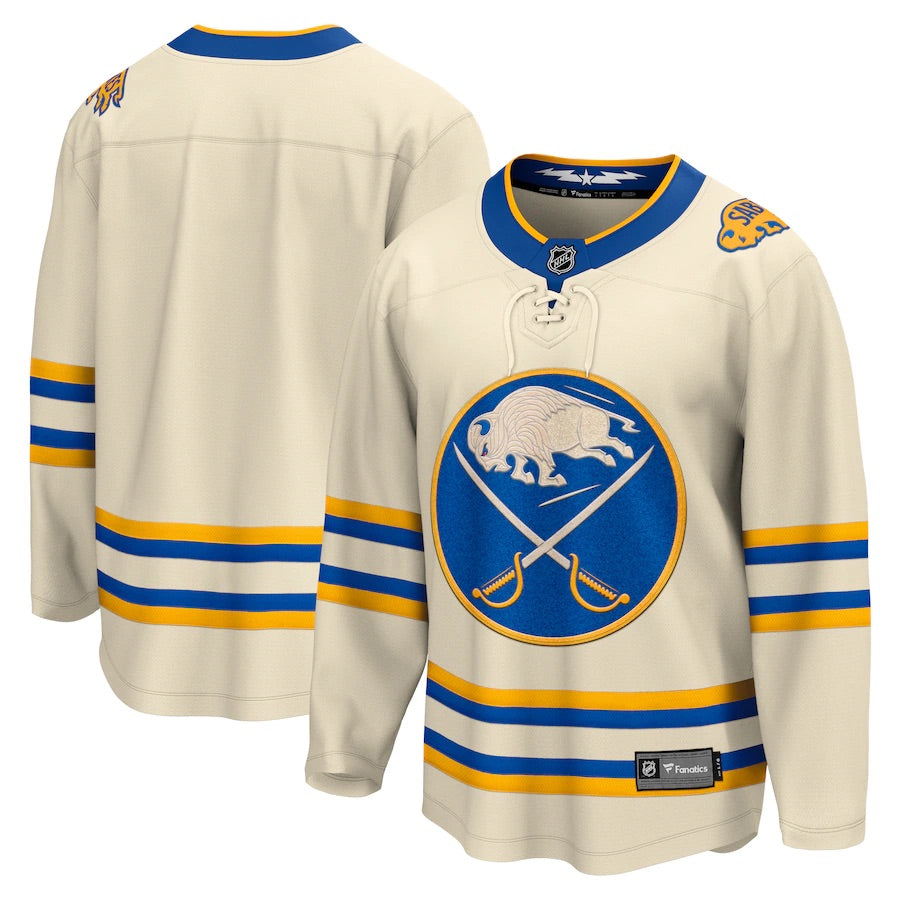The photograph showcases what appears to be antique NHL jerseys of the Buffalo Sabres, depicted from both the front and back views. The back view is positioned on the top left, and the front view is on the bottom right against an empty white backdrop. These primarily beige-white jerseys are adorned with distinctive stripes along the sleeves and waist, featuring a sequence of yellow, blue, white, blue, and yellow. The front of the jersey prominently displays a blue circle with a yellow outline, containing a white buffalo and two crossed sabers with gold handles. The neckline has a blue border accented with yellow, and there are ties at the top for fastening. Additionally, the shoulder features a yellow buffalo with the word "Sabres" inscribed on it. The color palette includes shades of blue, yellow, white, black, and gray.